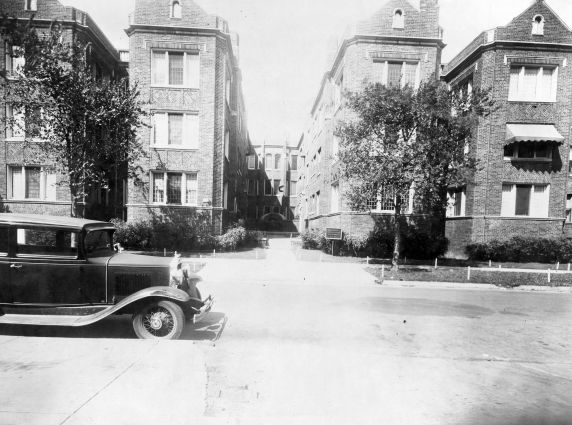This is a very old, black-and-white photograph depicting a street view of a symmetrical, multi-story brick residential complex with classic townhouse architecture. The image, likely taken in the early 1900s, features a black car parked by the curb on the left side, indicating early automotive technology. The complex showcases tall buildings with numerous windows, arranged in a symmetrical fashion that includes evenly spaced trees and grass along the sidewalk. A narrow alleyway is visible in the center of the photograph, leading to a small courthouse and presumably the lobby of the structure. The overall clarity of the image is very sharp, displaying no text or numbers, and it was clearly taken on a bright and sunny day. The composition suggests the photographer was standing directly in front of the buildings, focusing on their architectural symmetry and the serene street setting.